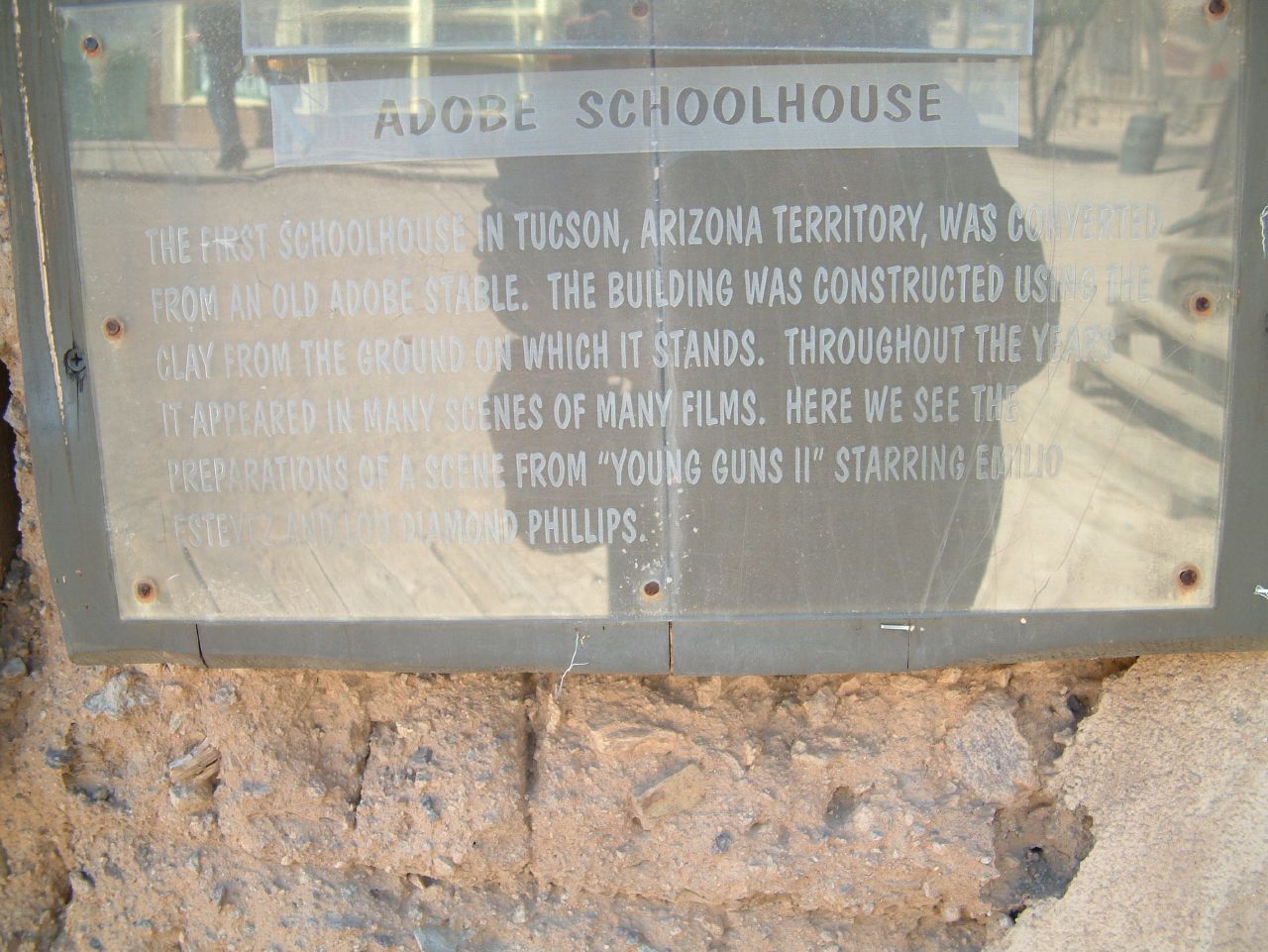This photograph showcases a plaque mounted on a clay-brown rock, commemorating the Adobe Schoolhouse, the first schoolhouse in Tucson, Arizona Territory. The schoolhouse, originally converted from an old adobe stable, was constructed using clay from the ground on which it stands. Over the years, it has appeared in various film scenes, including a prepared scene from the movie Young Guns 2, starring Lou Diamond Phillips and Emilio Estevez. The plaque itself is a silver reflective material with an all-capital white font inscription, bordered by a wooden frame and secured with rusty screws. Notably, the plaque includes a clear plastic cover and displays the reflection of the photographer and some old wooden stairs in the background, indicating it is part of a historical site that can be visited by tourists.